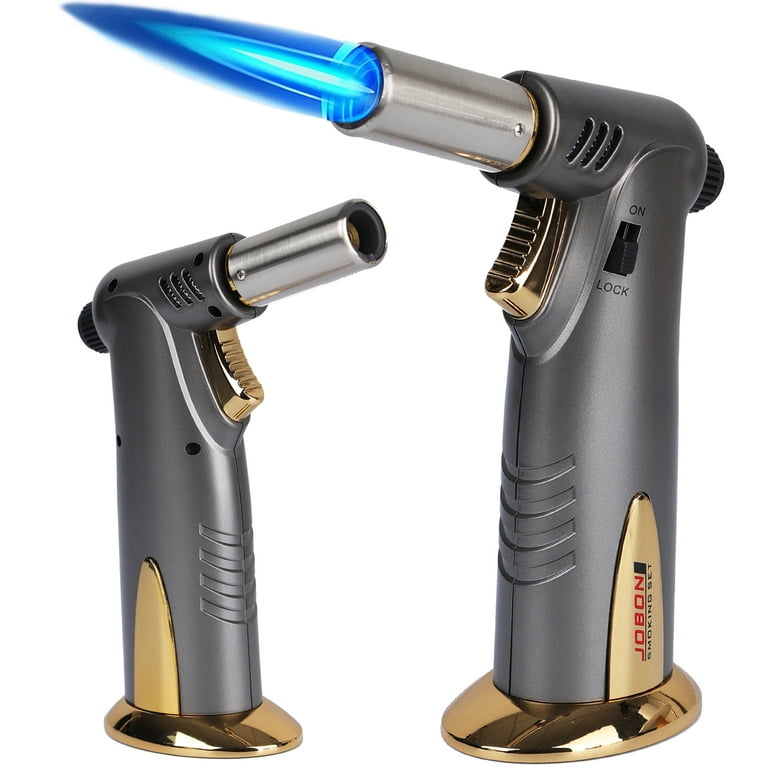This detailed product photograph captures two blowtorches prominently displayed against a white background, likely intended for a web sale. Both blowtorches share identical bronze-colored bases and feature sleek silver nozzles with gold or brass colored trimming. The smaller blowtorch, located on the left, has its nozzle pointed to the right, while the larger one on the right displays a striking blue flame emanating from its nozzle, which points to the left. Each blowtorch showcases an on-off switch and a trigger mechanism for handling. The larger model is explicitly marked with "Jobon Smoking Set," indicating the brand and product name.